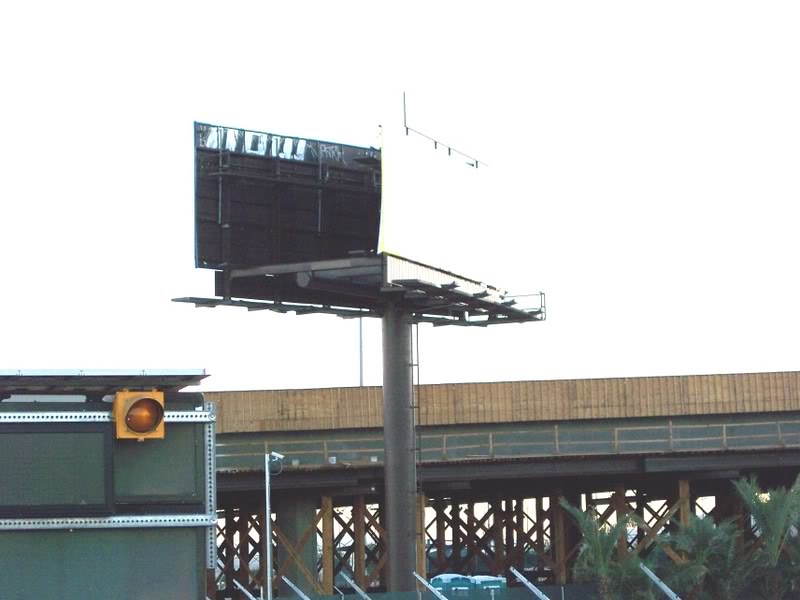In this photograph, we see a picturesque green bridge, characterized by its wooden railings and a maintenance walkway situated just beneath them. The bridge is supported by green concrete pillars and further reinforced with wooden beam cross sections, providing both aesthetic charm and structural integrity. Dominating the foreground, a metal billboard mounted on a single, sturdy steel pillar displays the faded and torn remnants of the word "NOW," and has been defaced with graffiti. Affixed to this pillar, several street lights are angled downwards, casting light onto the area below. To the left, either a segment of the bridge or an adjacent building features a yellow caution light, adding a touch of practicality to the scene. At the base of the billboard pillar, two porta-potties are situated, adding a utilitarian element to this urban landscape.